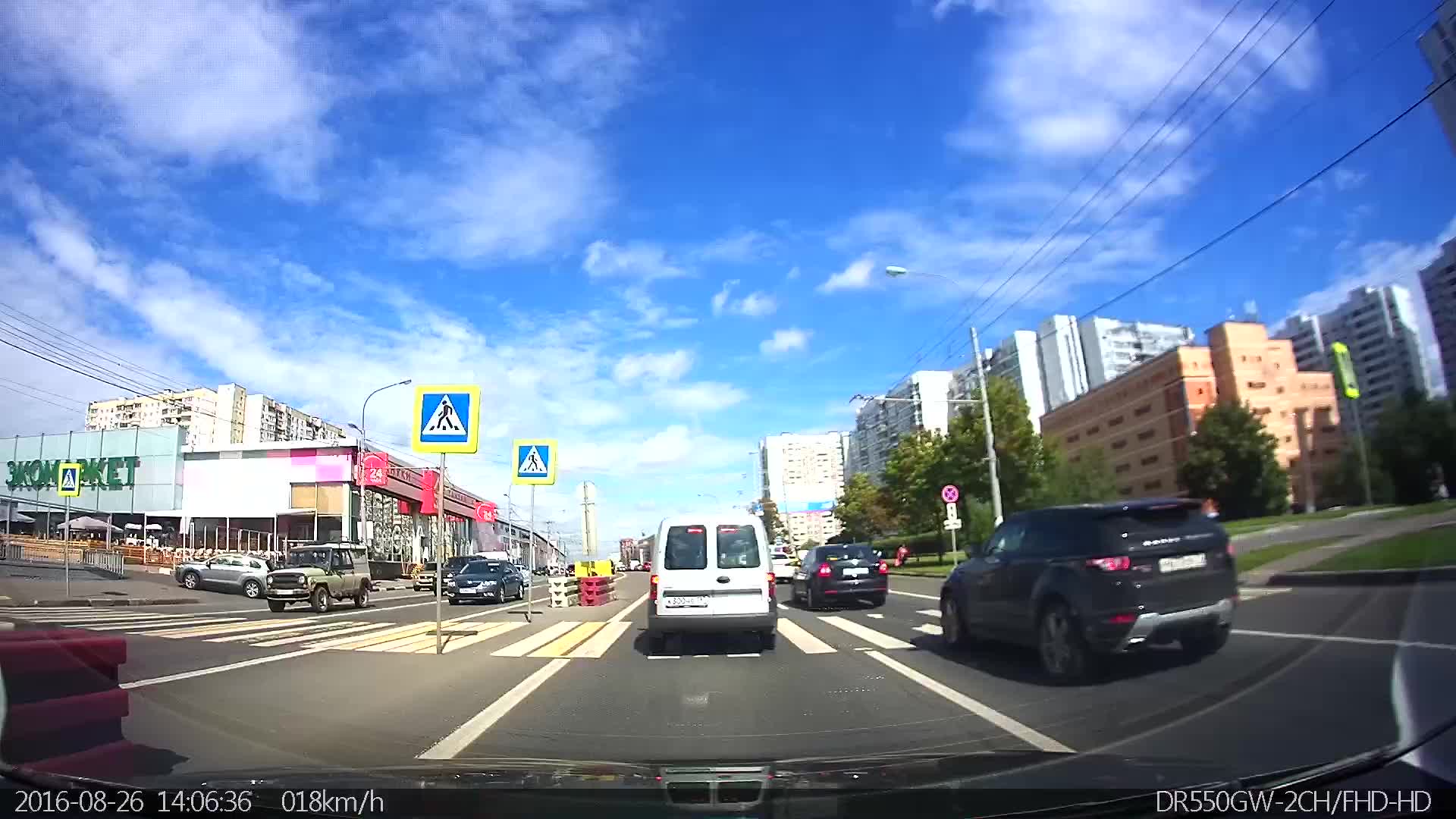This is a detailed photograph captured through the windshield of a car, showing a bustling urban street scene. The road in the center extends from the bottom of the image towards the horizon, featuring two lanes on the right side and several more on the left. The road is black asphalt with distinct white lane markings. On the lower left corner of the image, the timestamp "2016-08-26, 14:06:36" is visible, along with "018KM/H," indicating the speed of the car. The lower right corner displays "DR550GW-2CH-FHD-HD."

In the foreground, a white van with rectangular back windows is situated in one of the lanes, while a black SUV with a silver brand emblem is seen in the adjacent lane. The traffic is heavy, with cars moving in both directions. Road signs are present on the central divider; one notable sign is square with a white triangle and features a pedestrian figure, likely indicating a crosswalk near an actual crosswalk.

On the right side of the road, several large office buildings stand next to a green strip of grass, alongside power lines on poles. A parking garage and a stop sign are also noticeable on this side. To the left, there is a one-story market building with possible lettering "3 Con or Co Market," and behind it are additional office or apartment buildings.

The photograph depicts a clear day with a blue sky dotted with thin cumulus clouds, offering a snapshot of daily urban activity.